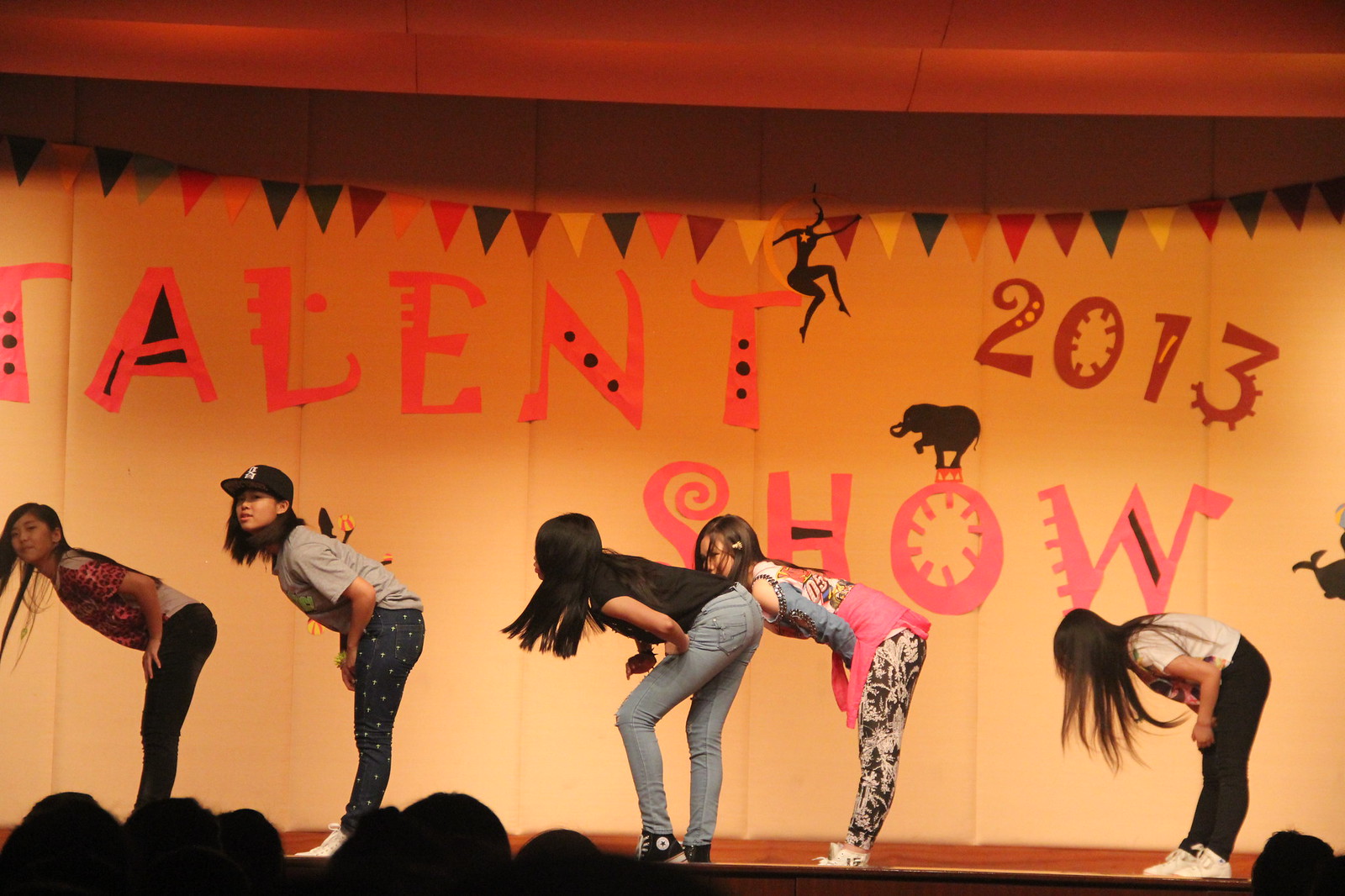This is a color photograph capturing a Halloween-themed performance on stage titled "Halloween 2023 Show," as stated in orange, black, and red text above the backdrop. The stage is adorned with diverse shades of orange, black, red, and brown, adding a festive vibe. Five performers, girls or young women, are clad in pink, white, black, blue, and polka-dotted costumes, with one sporting a noticeable hat. Positioned to the left, middle, and right of the stage, the performers are bent at the hips, all facing left in synchronized motion. In the background, additional elements like an elephant and a dancer appear as black silhouettes, and colorful painted banners adorn the top part of the stage. The scene also features the silhouettes of audience members in the foreground, slightly obscuring the lower part of the stage.